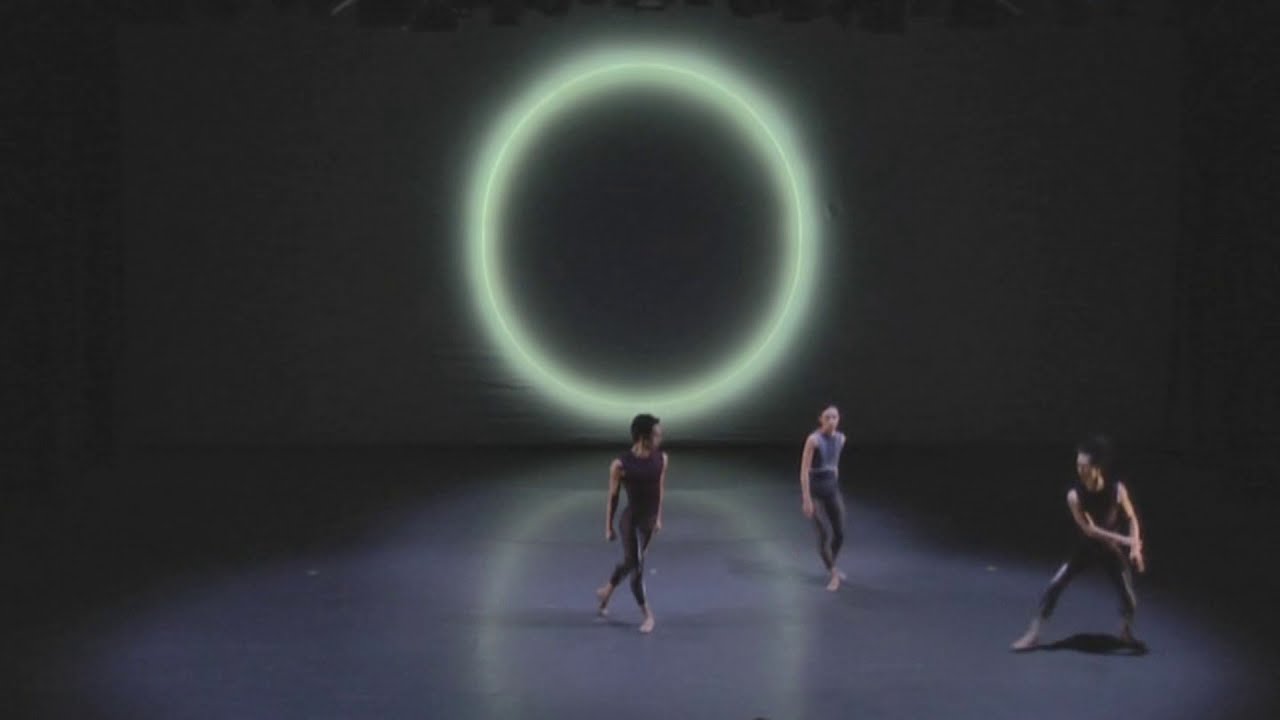This photograph depicts an indoor setting where three dancers are engaged in a practice session on a smooth, dark gray stage floor. The stage itself is predominantly dark with areas cast in shadow, except for a centrally illuminated, bell-shaped region. On the left side of this illuminated area stands a male dancer; at the center is a female dancer; and on the right side, another male dancer. The back wall is almost black and features a large, slightly grayish-green illuminated circle, which serves as the primary light source in this abstract environment. The dancers' reflections and the light from the circle can be seen on the stage floor. The dancers are in motion, dressed in athletic, yoga-style clothing. The central dancer, a male, is captured mid-pose with one leg in front and one behind, wearing a sleeveless dark purple shirt and tight pants, and is oriented towards the right side of the image. The female dancer in the middle is wearing a light sleeveless top with gray leggings, facing the first dancer with her back to us. The dancer on the right is executing a dynamic pose, with legs apart, his head turned towards the central dancer, while his right arm extends forward and his left arm reaches back.